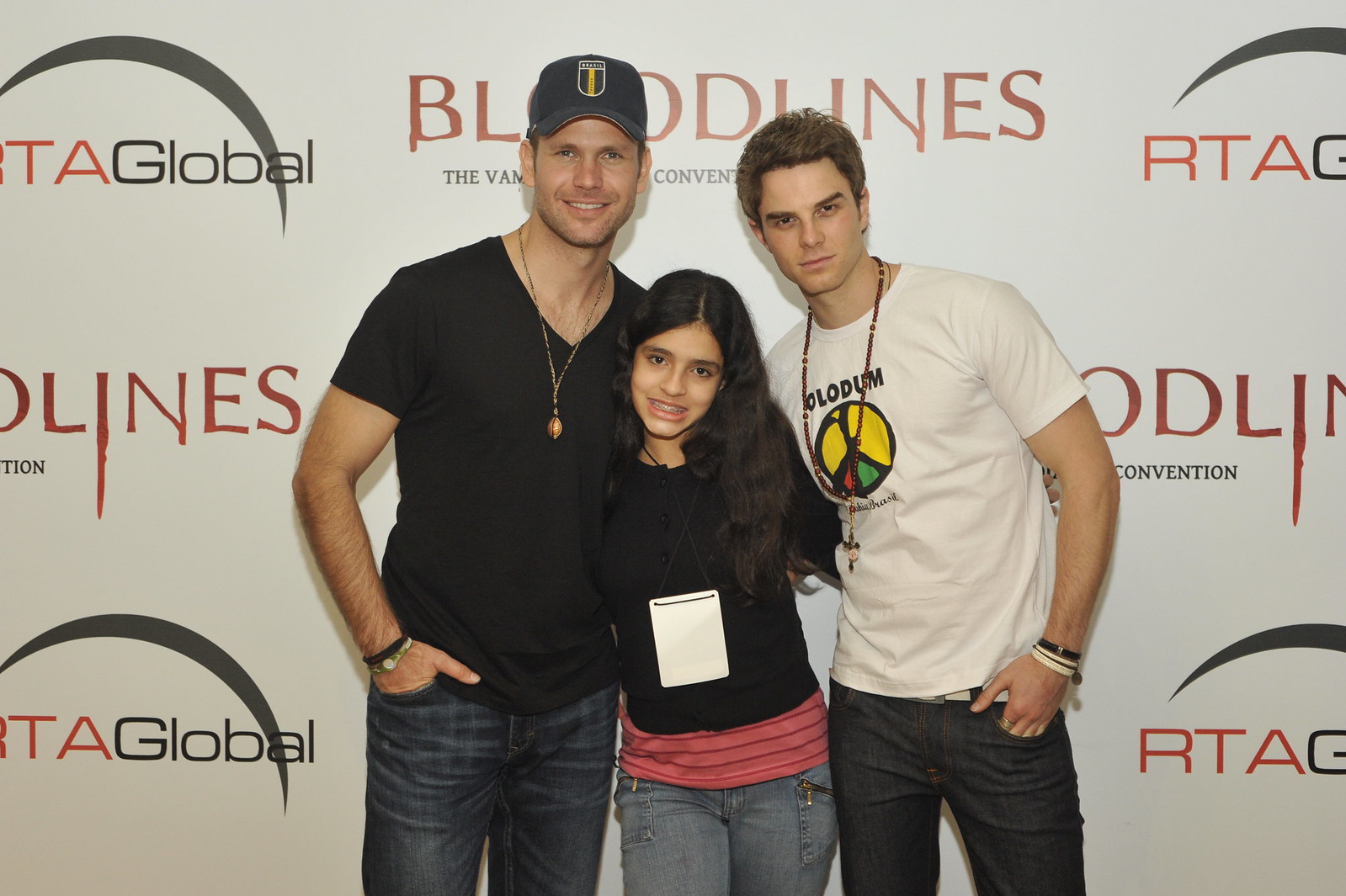The image features two men and a young woman standing against a white background adorned with repeated patterns of the words "Bloodlines" and what appears to be "RTA Global," accompanied by arching lines. 

On the left, there is a Caucasian man with dark eyes and stubble, wearing a black cap with an emblem. He is smiling and dressed in a black v-neck t-shirt, blue jeans, and a silver and bronze necklace. His right hand is casually placed in his pocket.

In the center stands a young Caucasian woman with long dark hair. She wears a black shirt over a pink shirt that peeks out at the bottom, and blue jeans. A lanyard with a white badge hangs around her neck. She has a warm smile, her head tilted slightly to the right as she leans towards the man on her left.

On the right is another Caucasian man with dark hair and eyes, dressed in a white t-shirt featuring a peace sign. He also wears a round necklace with a cross and bands on his wrist. His right hand is in his pocket, and he is angled slightly towards the woman in the center. All three are smiling and appear relaxed.